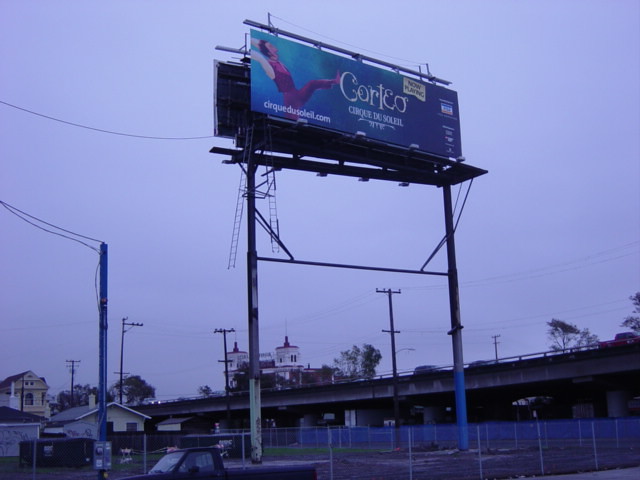This photo features an image of a billboard captured in a distinctive blue-tinted tone, as though a blue filter was applied. The billboard, oriented towards the lower right side due to the camera angle, prominently displays the word "CORTEO" in white font. Beneath it, although somewhat difficult to read, it appears to attribute the production to Cirque du Soleil. To the left of the billboard stands a person dressed in a vibrant red vest, energetically lifting both their arms and extending one leg straight in front of them, adding a dynamic and spirited element to the scene.